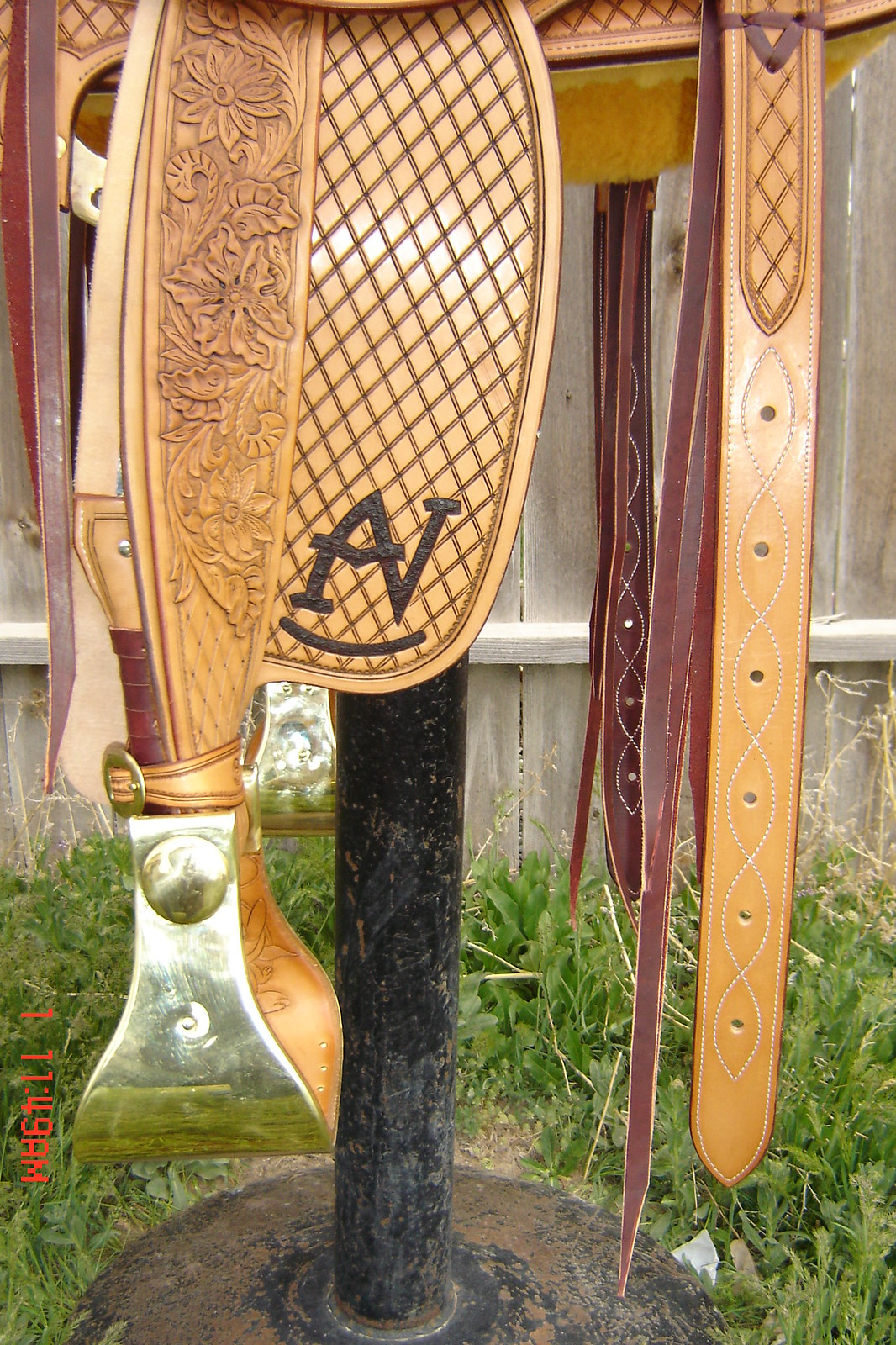This outdoor, daytime photograph focuses on the detailed lower half of an ornately decorated, light tan saddle resting on a heavily worn black stand with a circular base. The saddle, made of brown leather and clearly well-maintained, features intricate tooling with cross-hatched designs, flowers, and swirls. Prominently visible are the initials "A.V." stamped in darker brown leather with a small rocker detail beneath them. The polished metal stirrups, described as both silver and gold with a leather interior, dangle from the saddle's ornate leather straps, which are adorned with engraved floral patterns. Additional tan straps with decorative stitching hang to the right, suggesting their use for securing the saddle to a horse. The scene is set against a backdrop of green grass and a rustic wooden fence.